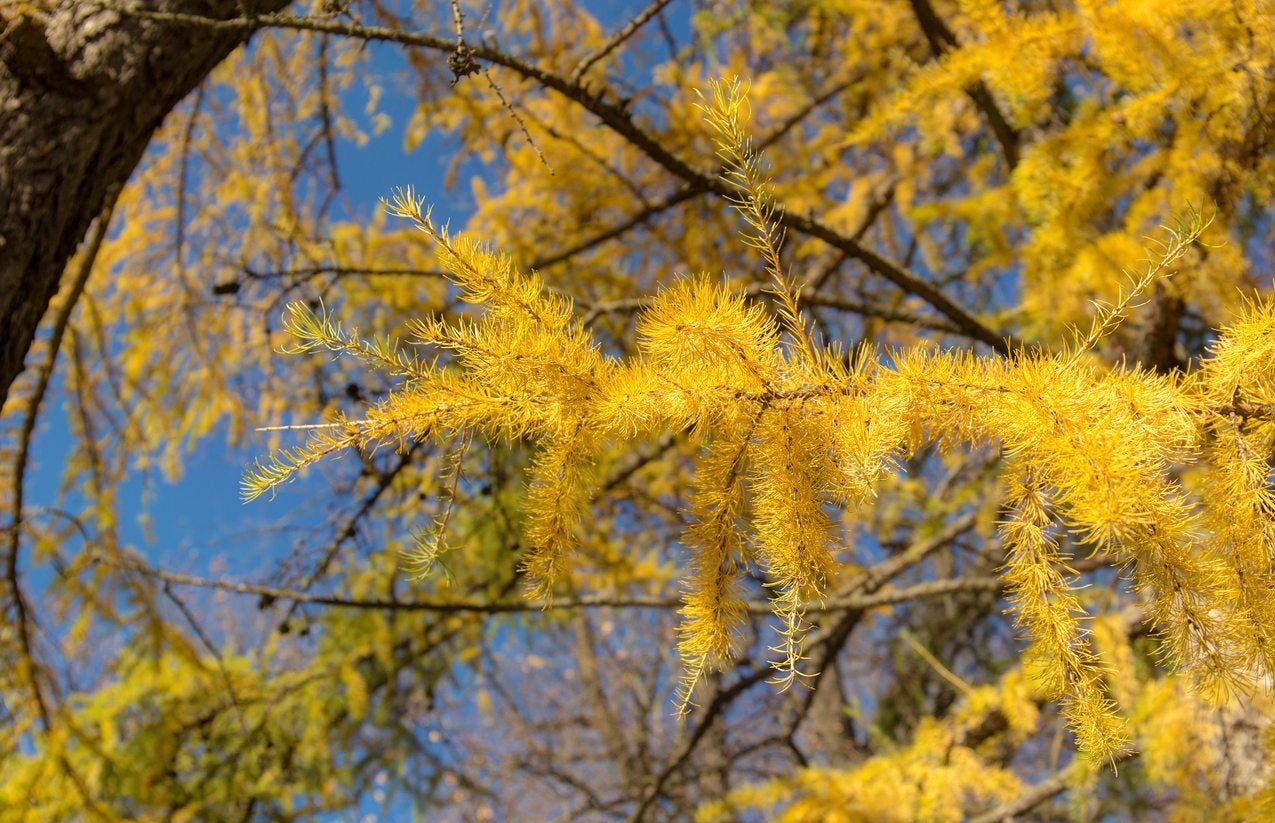This vibrant, high-quality landscape photo captures the essence of autumn on a bright, sunny day. The image features a close-up view of a tree, likely a pine, with branches adorned with striking, yellow-gold pine needles cascading from the right side of the frame. The tree's trunk peeks in from the top left corner, grounding the image against a brilliant, clear blue sky. As you gaze upward, the intricate details of the pine needles, resembling thin, spiky thistles, create an intriguing contrast with the sky. The vivid colors and depth, with some branches in sharp focus and others blurred in the background, highlight the serene beauty of this fall day.